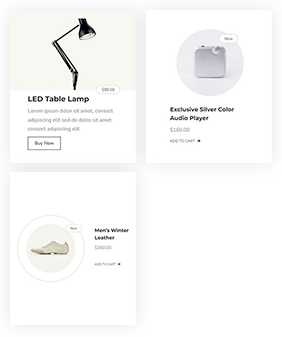The image depicts a small screenshot from what appears to be an e-commerce site. The layout comprises three small rectangular product images set against a predominantly white background, with a pale gray backdrop. There is no visible navigation bar or additional site information. 

In the top left corner, there is an image of a modern LED table lamp featuring a hinged arm for adjustable lighting. Below this image is some descriptive information, likely detailing the product features.

Beneath the lamp image, there is a white rectangular block showcasing a circular inset. Within this circle is a stylish white leather shoe, with the tip of the shoe pointing to the left. 

In the top right corner, another white rectangular block features a small square object placed inside a gray circle. Below this image, text reads "exclusive silver color audio player."

Though the text and prices are too small to decipher clearly, it appears that each product listing includes pricing information and options to purchase or add the items to a shopping cart.